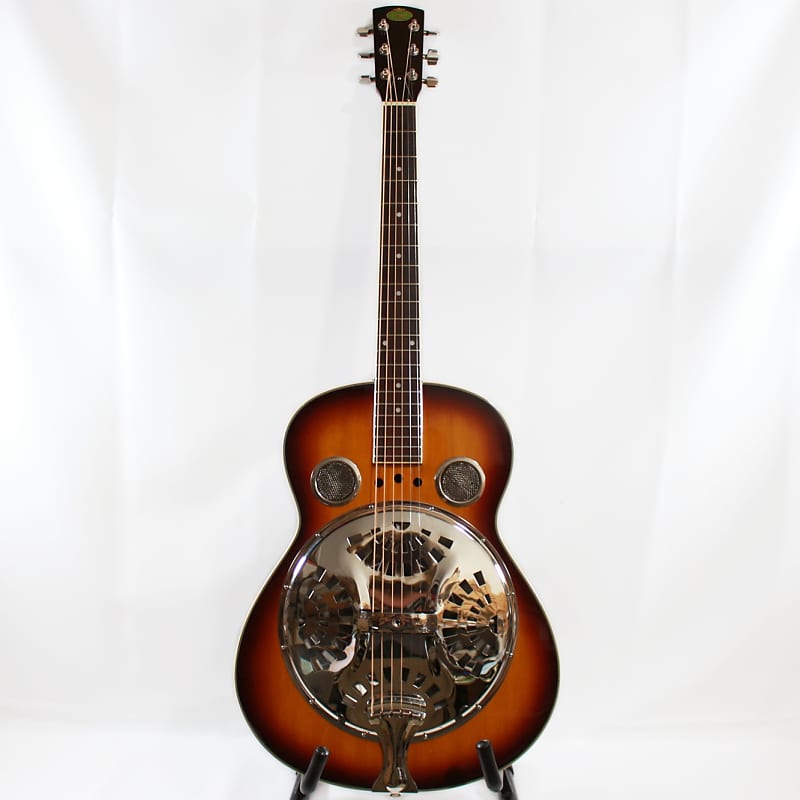The photo features a striking brown guitar with a contrasting blend of dark edges and a lighter interior, presenting a gradient of burnt to yellowish wood tones. The guitar is positioned upright on a stand, which is partially visible at the bottom, and is directly facing the camera, with the neck pointing upwards. The body of the guitar is adorned with a shiny, chrome plate that covers a significant portion of the center, embellished with rectangular holes reminiscent of a banjo. Additionally, there are two small, circular chrome-bordered areas located near the top part of the body, flanking the strings. The whole setup is against a white background that appears to be a fabric or heavy plastic sheet, exhibiting noticeable folds, wrinkles, and some glary reflections on both sides.